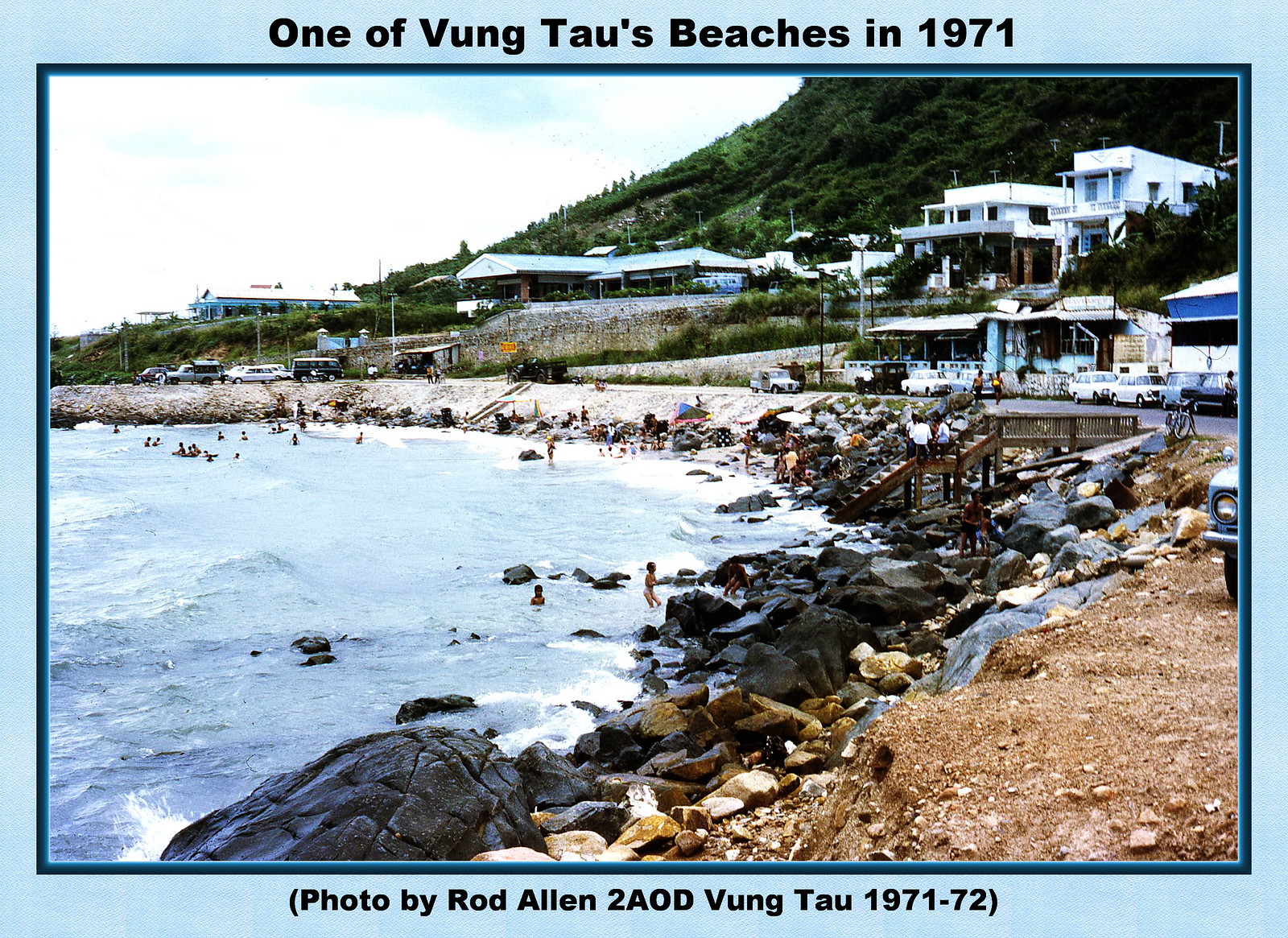This photograph, bordered in light and dark blue, depicts one of Vung Tau's beaches in 1971, as noted at the top of the image. The lower part of the border states, "Photo by Rod Allen 2AOD Vung Tau 1971-72." The picture captures a coastal town with a serene yet slightly nostalgic atmosphere, characteristic of old-time photos. The beach curves from the bottom left to the middle left in an arc, with numerous black rocks and shells scattered along the shoreline.

In the foreground, people are seen enjoying the water, while on the left side, cars drive along a road that wraps around the beach. A staircase pier leads up to the road, connecting to a parking area filled with light blue buildings. Further to the right, several multi-story houses, which appear to be beach houses, are nestled on a hillside. Above these buildings, a hilly, mountainous area covered in lush green trees and bushes stretches across the upper right corner of the photo, adding depth to the scenery. The main colors that dominate this image are the green of the mountains, the blue of the water, the gray of the stones, the brown of the beach sand, and the white of the buildings, creating a harmonious coastal scene.